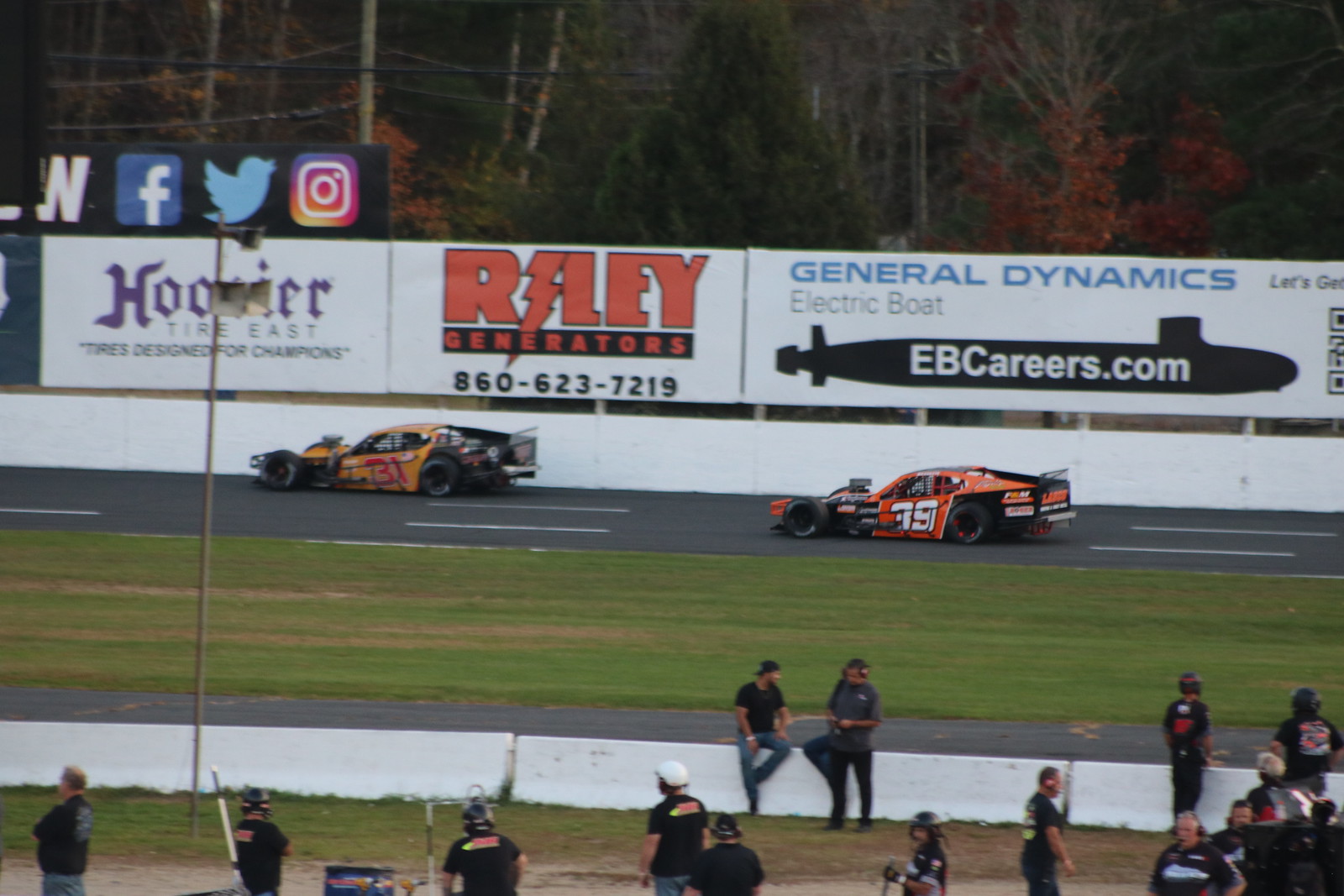In this vibrant image captured at dusk, two race cars, one a vivid orange and the other a yellowish-orange, speed around a racetrack. The car with the red number 31 and the other with the white number 35 are competing fiercely on the gray and black track lined with white markings. Surrounding the track is an inner ring of lush green grass. In the foreground, several men in dark shirts and ball caps or helmets stand attentively, likely officials or crew members. 

Adding to the dynamic atmosphere, colorful signs embellish the wall bordering the track, including prominent ones that read "General Dynamics Electric Boat EBCareers.com," "Ray Generators," and "Hoosier Tire East," adorned in purple, orange, and blue hues. Beyond this wall, another barrier backs onto a wooded area showcasing a tapestry of tree leaves in various autumn colors: green, red, and orange. The image subtly hints at the waning light of dusk, casting a warm glow over the entire scene, from the men seated on the distant wall to the lively forest backdrop.